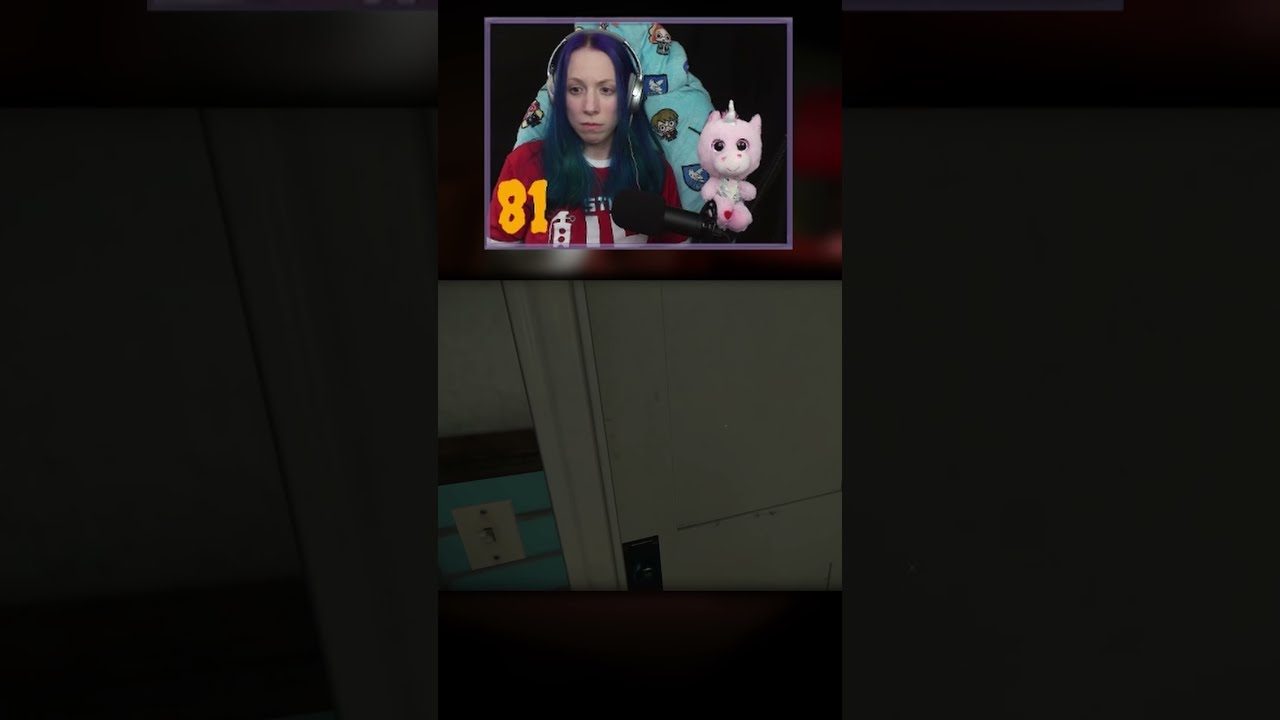The image is divided into three vertical sections, with the first and third sections showing darkened, close-up versions of the central picture. The central section is further split into three horizontal portions. The top portion features a woman in a purple rectangular frame. She has long hair dyed in shades of blue and green and is wearing silver over-the-ear headphones. The woman, dressed in a red shirt with white patterns, sits on a blue chair adorned with cartoon figures. Positioned to her right is a pink stuffed animal resembling a unicorn. In front of her is a black microphone, and the number "81" is displayed in yellow at the bottom left corner of the purple rectangle. The middle horizontal section appears to be a screenshot from a video game, showing a white wall with a blue lower half and a white door with a black lock on the right side. The bottom section is dark, with a brown and black background. The left and right thirds of the overall image feature enlarged, grayed-out close-ups from the video game section, creating a blurred effect on the sides.